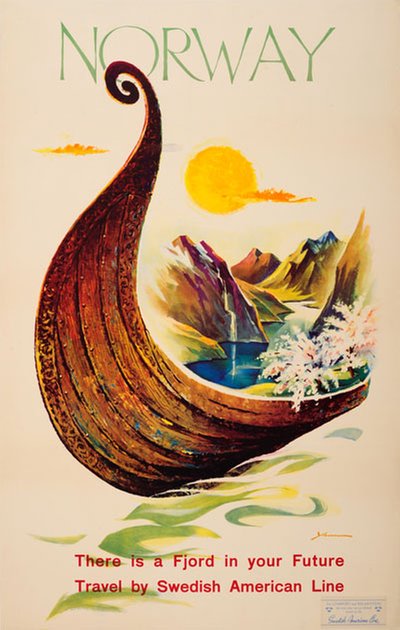The image resembles an advertisement poster with an off-white beige background, giving it an aged appearance. At the top, in striking green capital letters, it reads "Norway." Below this text, there is a vibrant depiction of a yellow sun surrounded by small, orange clouds. The centerpiece of the image features a gondola-like boat crafted from dark wood with a spiraled tip at its prow. The interior of the boat creatively represents the Norwegian landscape with abstract elements: golden-brown mountains, a flowing river or stream, and a white flowering tree or bush on the right. Swirling green patterns at the bottom of the boat suggest water. At the bottom of the poster, in bold red letters, the slogan reads, "There is a fjord in your future. Travel by Swedish American Line."